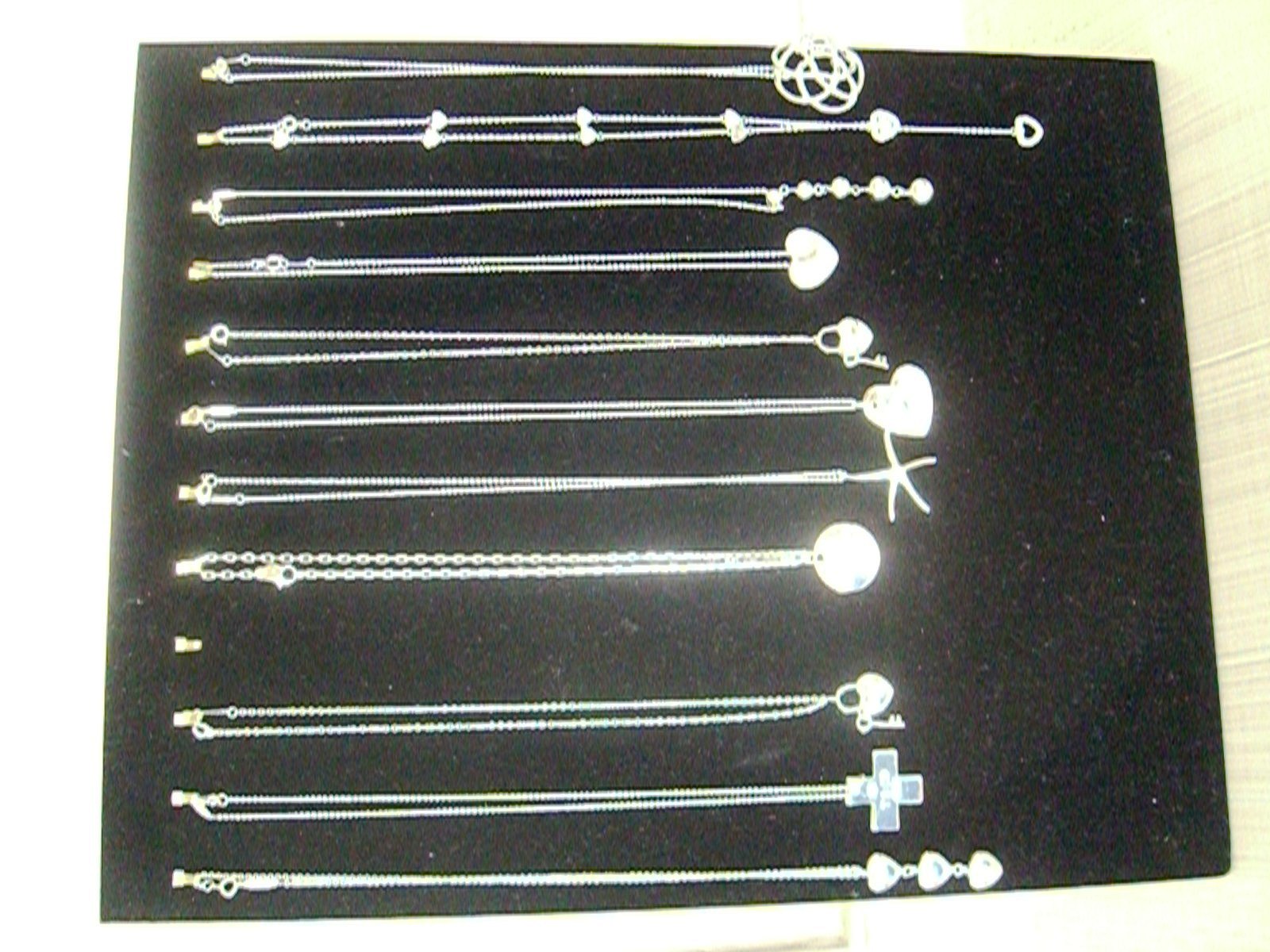The image features 11 silver necklaces displayed horizontally against a soft, black suede-like background, which is set on a white surface. Each necklace is suspended from small hooks, though the fourth spot from the bottom is empty. The necklaces vary in design, including charms such as linked hearts, a square cross with equal arms, heart-shaped locks with tiny accompanying keys, a plain silver pendant that could be engraved, a five-armed starfish, and multiple designs featuring circles and beads. The details of the necklaces and the charms, including hearts, a horse, two gems, a pendant with beads around it, and several geometric shapes like triangles, are somewhat obscured by light reflections. Despite the unclear image quality, the display is likely aimed at a younger audience, perhaps teenagers, given the affordable appearance of the jewelry and the playful nature of the designs.